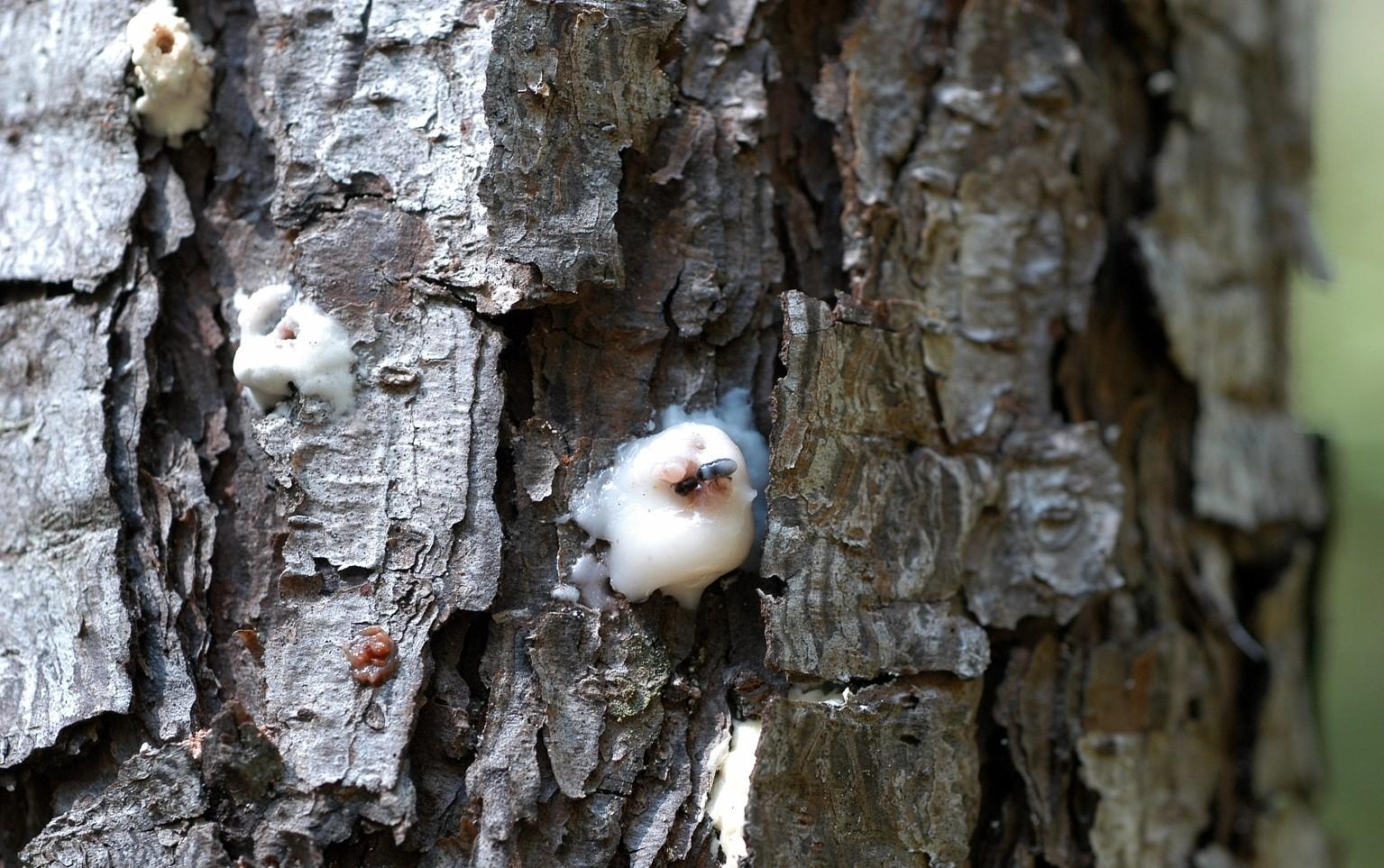The image presents a detailed close-up of an aging tree trunk with gray-brown bark, textured and weathered. Prominently featured on the bark are several white, foamy, marshmallow-like blobs that appear to be a type of fungus. These patches of fungus are scattered in at least three distinct sections: one in the upper left corner, another diagonally down towards the middle of the trunk, and a central one almost dead center on the tree. The central blob has a small black bug, possibly an ant or fly, burrowing into it, adding a dynamic element to the otherwise still scene. Smaller brown blobs are also visible towards the bottom left corner. The lighting suggests the photo was taken during the daytime, and the rectangular frame captures the horizontal expanse of the bark in sharp detail, while the right side of the trunk fades into a blur.